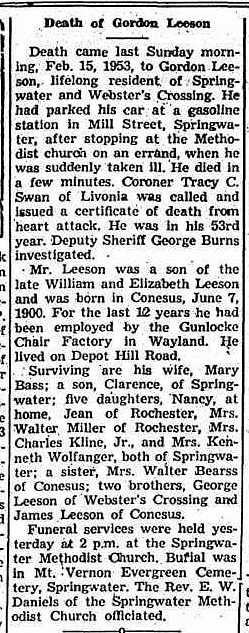This is a tall, rectangular screenshot from a newspaper article, displaying thin black borders and black text on a white background. The article is an obituary titled "Death of Gordon Leeson." It reports that Gordon Leeson, a lifelong resident of Springwater and Webster's Crossing, passed away on Sunday morning, February 15, 1953, at the age of 52 (in his 53rd year). After stopping at the Methodist Church on an errand, he parked his car at a gasoline station on Mill Street in Springwater, where he suddenly fell ill and died within minutes. Coroner Tracy C. Swan of Livonia confirmed the cause of death as a heart attack, and Deputy Sheriff George Burns conducted the investigation. Gordon Leeson was the son of the late William and Elizabeth Leeson, born on June 7, 1900, in Conesus. For the last 12 years, he had been employed by the Gunlock Chair Factory in Wayland. He lived on Depot Hill Road and is survived by his wife, Mary Bass, a son named Clarence of Springwater, and five daughters: Nancy, who remained at home, Jean of Rochester, Mrs. Walter Miller of Rochester, Mrs. Charles Klein, Jr., and Mrs. Kenneth Wolfganger. The article includes additional paragraphs below the provided text.